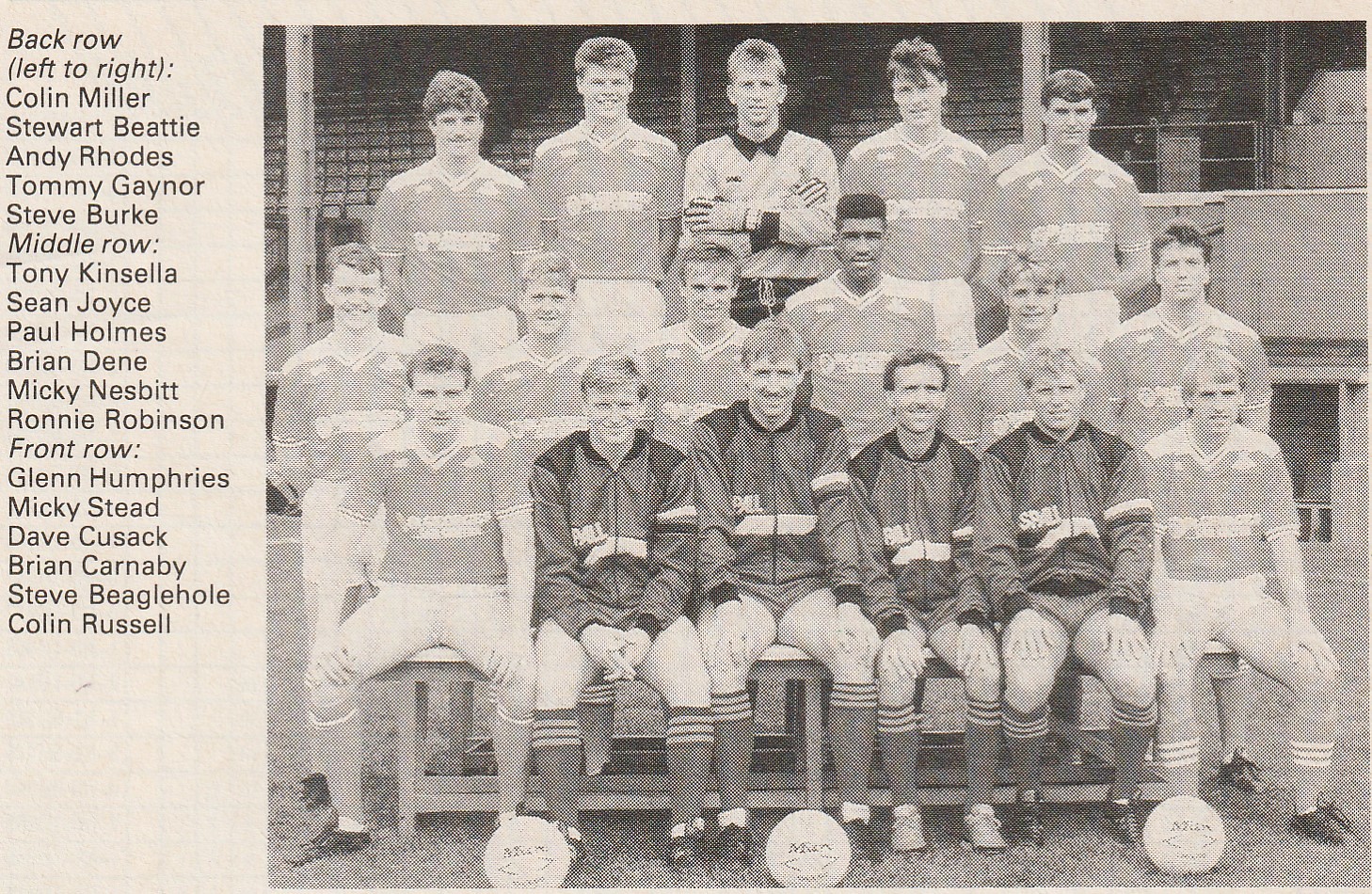This is a black and white photograph, possibly a newspaper clipping or a game day program, depicting a soccer team in a landscape layout. The image appears to be from the 80s or 90s, given its grainy and slightly blurry quality. The team is composed of all men, arranged in three distinct rows. The front row, with six players, is seated and has three soccer balls placed at their feet. The middle row of six players stands directly behind them, and the back row, also consisting of six players, is elevated, likely standing on something to add height. Most players are white, with one black player positioned in the middle row. All players are dressed in their team uniforms which include short-sleeved shirts with writing on the front and white shorts. To the left of the image, black text lists the names of the players by row: back row from left to right are Colin Miller, Stuart Beattie, Andy Rhodes, Tommy Gaynor, and Steve Burke. The middle row includes Tony Kinsella, Sean Joyce, Paul Holmes, Brian Denny, Mickey Nesbitt, and Ronnie Robinson. The front row features Glenn Humphreys, Mickey Stead, Dave Cusack, Brian Carnaby, Steve Beaglehole, and Colin Roussel.